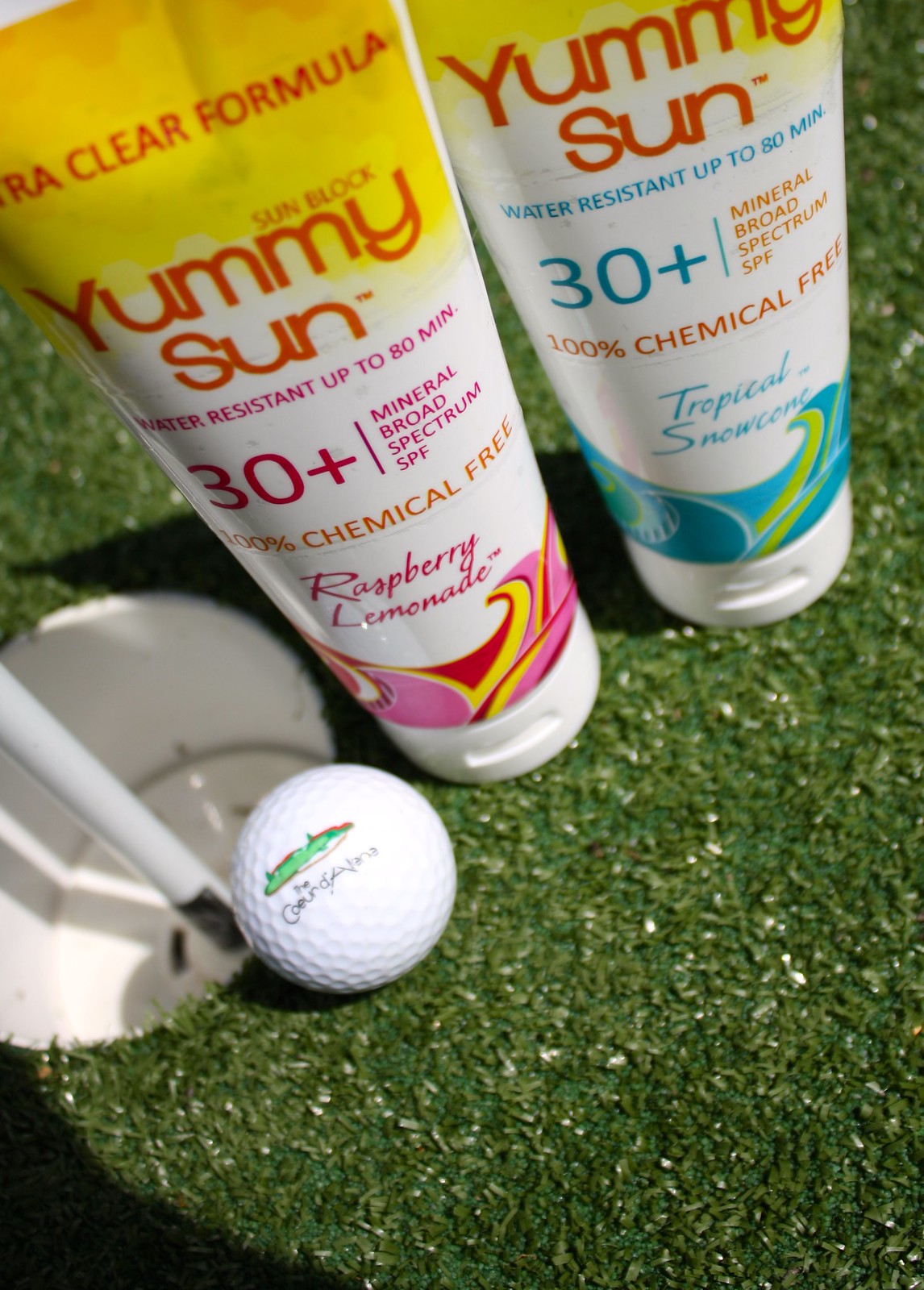This vertically aligned photograph captures a detailed view of various objects arranged on vividly green artificial turf, possibly situated on a golf course. At the lower left side of the image, a golf ball with some sort of green design and unreadable text is seen resting right next to a white cup-style golf hole, with a white flagpole emerging from it. Positioned prominently to the right, there are two plastic containers of sunscreen. The left container, with a pink and white design, reads "Yummy Sun Clear Formula" against a yellow background and is labeled "Raspberry Lemonade" scent. It also states key features such as "Water-resistant up to 80 minutes," "30+ Mineral Broad Spectrum SPF," and "100% Chemical Free" in red letters. The similar container on the right features a blue and white design and is labeled "Tropical Snow Cone" with identical sunblock attributes. The image, possibly part of an advertisement, reflects a bright, midday outdoor setting, meticulously showcasing both the golf-related and skincare products in vibrant, contrasting colors.